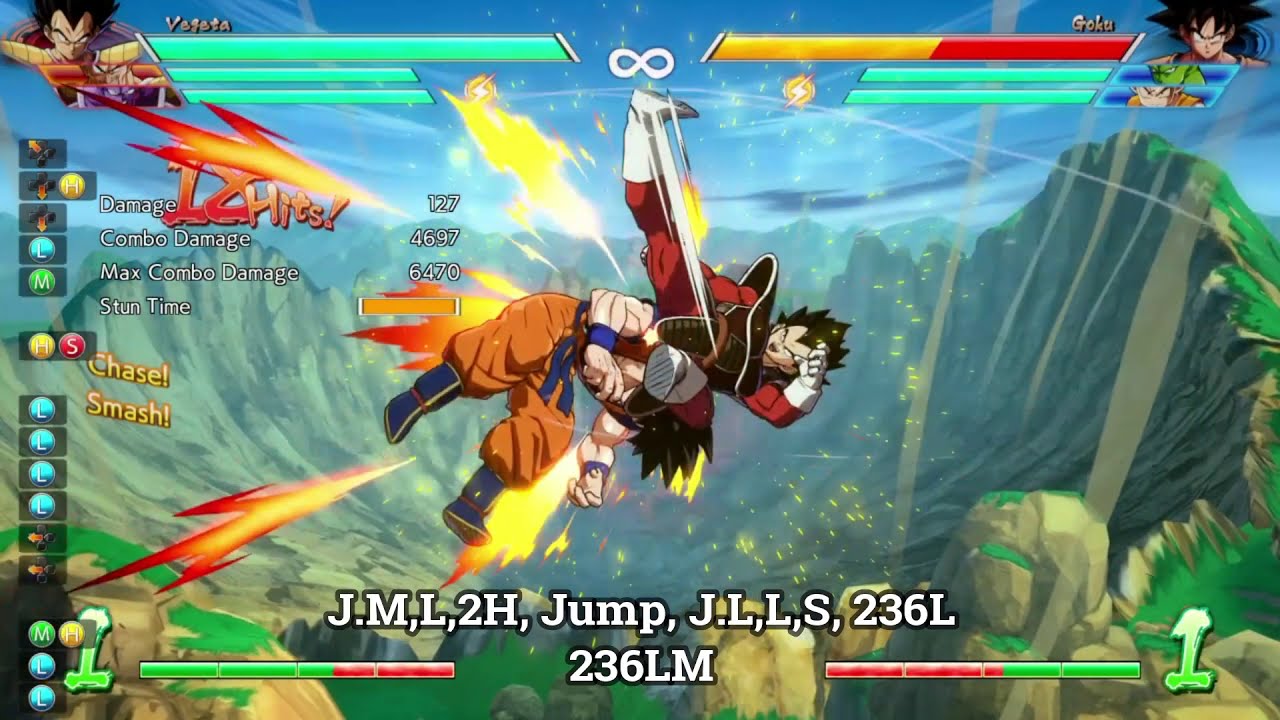This detailed screenshot depicts an intense moment between two iconic characters from the Dragon Ball Z universe, Vegeta and Goku, as they battle in a high-fidelity video game with graphics that closely resemble the anime's art style. Positioned in mid-air, Vegeta, clad in a red suit with white boots, a shoulder guard, and chest armor, is executing a powerful upward kick aimed at Goku's head. Fire sprouts from Vegeta's foot, emphasizing the force and impact of the strike. Goku, wearing his signature orange attire, is engulfed in flames due to the severity of the attack.

In the background, a crater indicates prior destruction, hinting at the ongoing battle’s intensity. Above the characters, health bars with avatars indicate the status of each fighter, with additional team members visible and ready to join the fray. Text onscreen includes "18 hits" in red and yellow, denoting the number of strikes landed, and various game commands such as "J.M,L,2H,J,J.L,L,S,236L" and "236LM" displayed at the bottom. This advanced Dragon Ball Z fighting game, reminiscent of titles like Street Fighter, showcases the dynamic and precise animation of the characters, capturing the essence of the anime in a modern gaming experience.